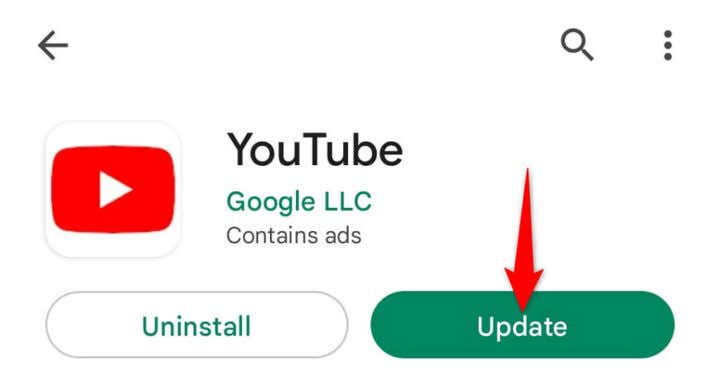The image is a screenshot of the YouTube app's page on the Google Play Store. At the top left, there is a grey back arrow. On the top right, there is a magnifying glass icon for search functionality, followed by three vertically stacked dots that represent more options. On the left side next to the back arrow, there is the YouTube play button icon, which is red with a white triangle play symbol in the center. Next to the play button, the text "YouTube" is written, followed by "Google LLC" in green letters. Below that, in grey text, it says "Contains ads." Below this information, there are two buttons: on the left, a white button with green text that says "Uninstall," and on the right, a green button with white text that says "Update." There is a red arrow pointing at the "Update" button.